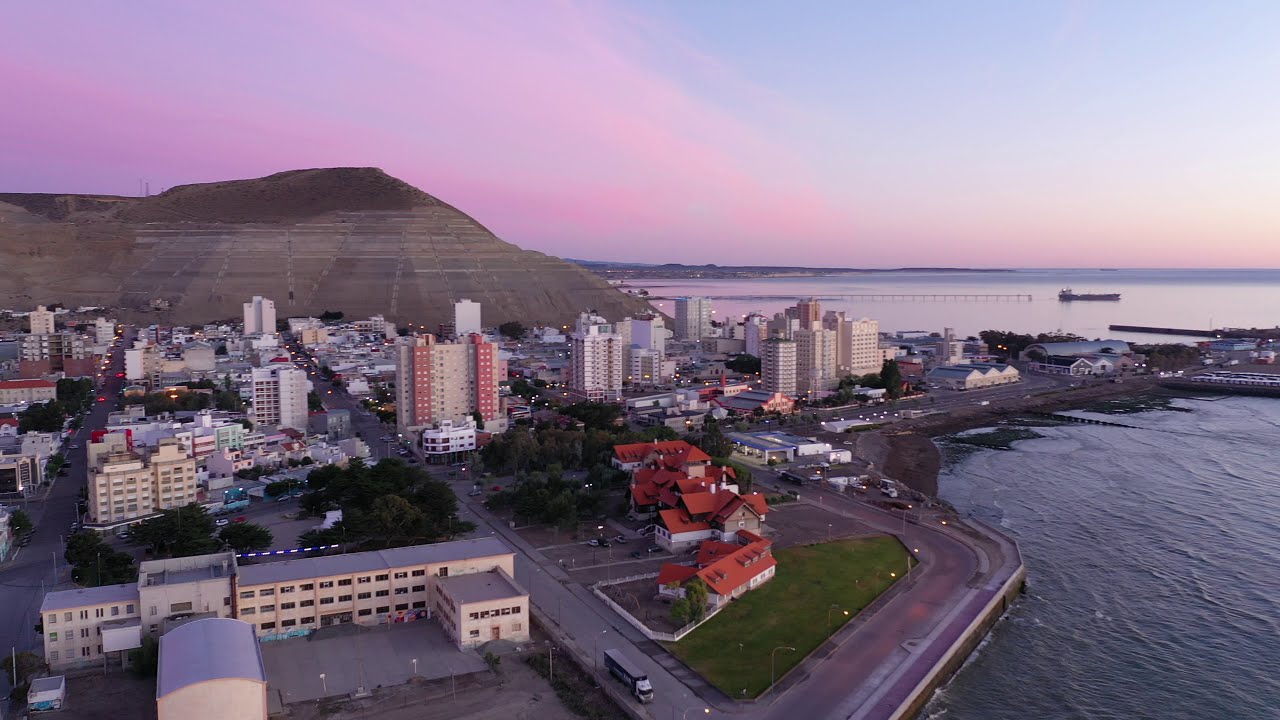This stunning photograph captures a bustling coastal city at twilight, either dawn or dusk, with a vibrant sky painted in shades of pink, purple, and blue. The cityscape is rich with details, showcasing numerous tall and short buildings, possibly apartments, hotels, or condos, some adorned with red roofs especially close to the water's edge. As the city lines the coast, a network of crisscrossing roads is visible, with a few vehicles navigating through them.

On the right side of the image, a vast expanse of water dominates, likely an ocean or a large bay, featuring a long pier jutting out into the inlet. A sizable cargo ship or container vessel is seen anchored in the distance. The left side of the photograph is marked by a prominent large hill or cliff, mottled in brown and tan hues, resembling a mining site or similar to the Diamond Head volcanic tuff cone found in Hawaii, adding dramatic contrast to the urban scene.

Overall, this richly detailed image highlights the serene beauty of a port city harmonizing with its natural geography, under a mesmerizing, colorful sky as the day transitions to night or dawn.